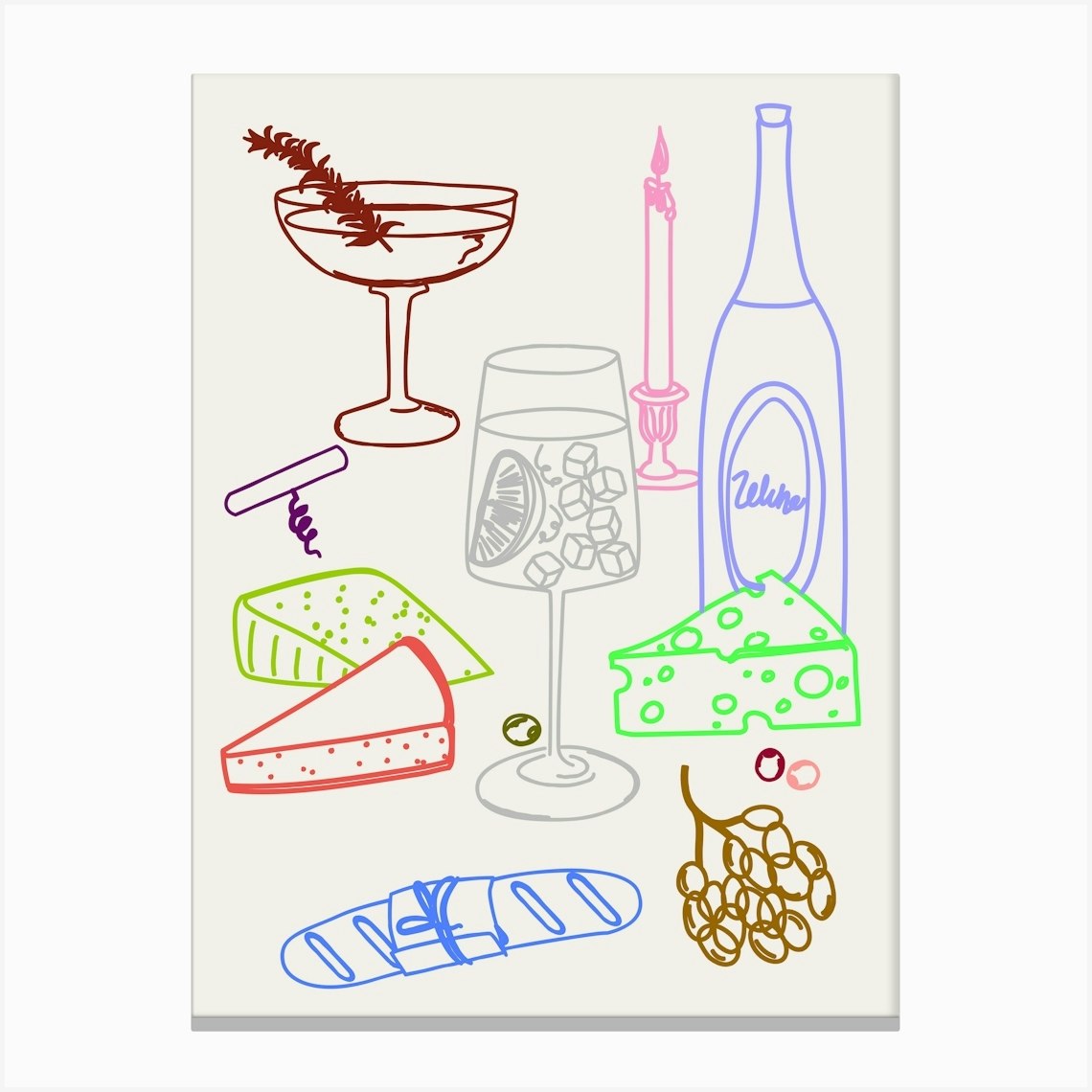The image is a detailed, colorful drawing on a white canvas with a gray line at the bottom. Central to the composition is a glass filled with liquid, ice cubes, and a slice of lemon, all outlined in grey. Surrounding the glass are various food items, including a piece of bread tied with a rope, stylized in blue, and clusters of brown grapes. To the left of the glass are three cheese slices: one red, one green, and another yellow-green shade, outlined differently for variety. To the right of the glass, there's another cheese wedge in a different green hue.

Alongside these items, another glass is depicted; this one holds a red liquid with what appears to be a feather or leaf garnish. A purple corkscrew is visible nearby. Above these, the drawing features a pink candle on a stand and a blue wine bottle. The entire arrangement is presented against a white background, with an assortment of colorful, outline-drawn food and drink items giving the image a vibrant yet simple charm.